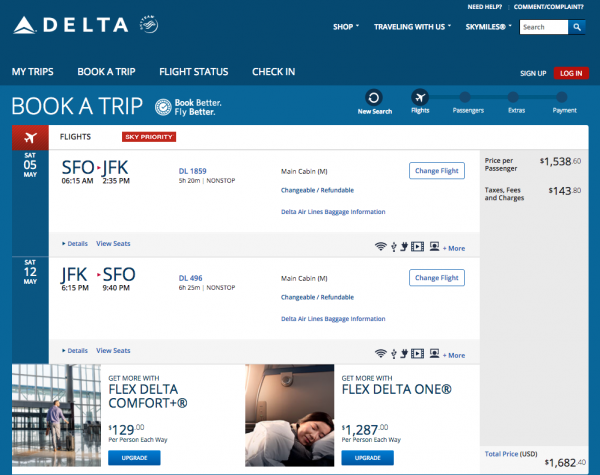The web page features a detailed layout centered around Delta Airlines. At the top of the page is the prominent Delta logo, set against a blue background with a triangle that has a fine line cutting through its base. On the far right side, there's a dropdown menu under the "Shop" section. Nearby, you'll find "Traveling with Us" and "SkyMiles," Delta's frequent flyer program that awards miles for each flight. Adjacent to these is a search bar. 

Above these options, there's a "Need Help" section for inquiries or complaints. Below the Delta logo on the left, several options are all capitalized: "MY TRIPS," "BOOK-A-TRIP," "FLIGHT STATUS," and "CHECK-IN." The main section features a message reading "Book Better, Fly Better" with a status indicator to the right, showcasing a plane in flight and offering a new search function for flights. Proceeding further down, you'll find sections for passenger details, extras, and payments.

The page displays two specific flight options in a column on the left, marked by a red background with a white airplane icon. The first flight is on Saturday, May 5th, from San Francisco (SFO) to New York (JFK), departing at 6:15 AM and arriving at 2:35 PM, totaling nearly five and a half hours of non-stop flight. It indicates the main cabin is changeable and refundable. There's also an option to click "Change Flight."

The second flight shown is on Saturday, May 12th, from JFK to SFO. Similar details are provided, including upgrade options to Delta Comfort and Delta One, with respective costs. 

On the right side, a gray column lists the price for passengers at $1,538, additional taxes and fees of $143, culminating in a total price of $1,682.40, clearly displayed at the bottom in blue U.S. dollars.